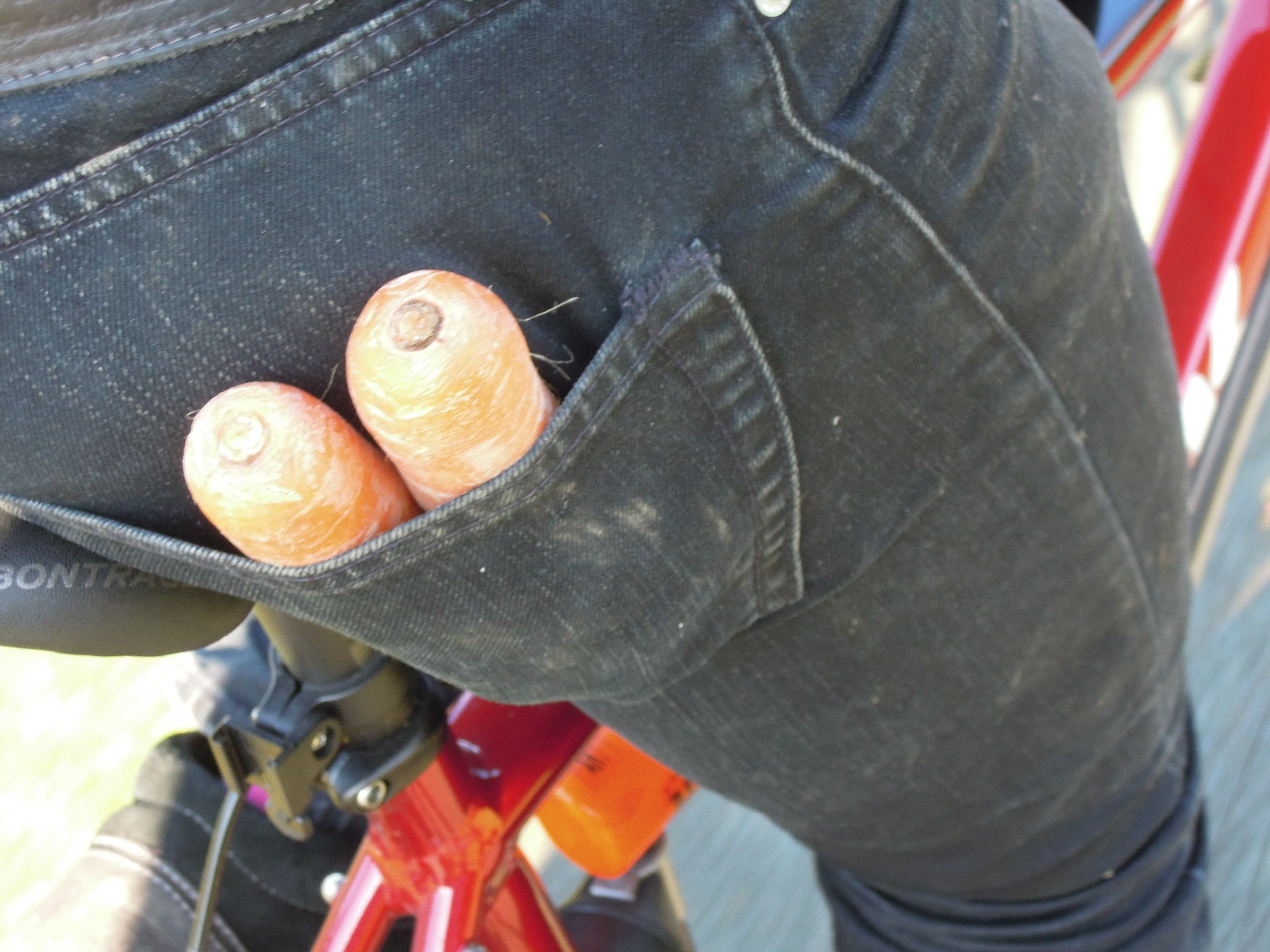The image is an up-close photograph of a person seated on a bicycle, primarily focusing on their lower half. The individual is wearing black or dark gray faded denim jeans, which appear slightly dirty and wrinkled, particularly around the knees. In the back right pocket of the jeans, there are two large, somewhat dirty carrots with white streaks and tiny hairs visible. The bicycle has a red frame, visible around the seat post area, and a black saddle. Also noticeable is an orange and black sports water bottle clipped beneath the frame. The scene is set outdoors on a streaked asphalt surface, and other details include the person's black boots with gray and white stitching, and the brake cables of the bicycle. The letters "O-N-T-R-A" are partially visible on the seat.